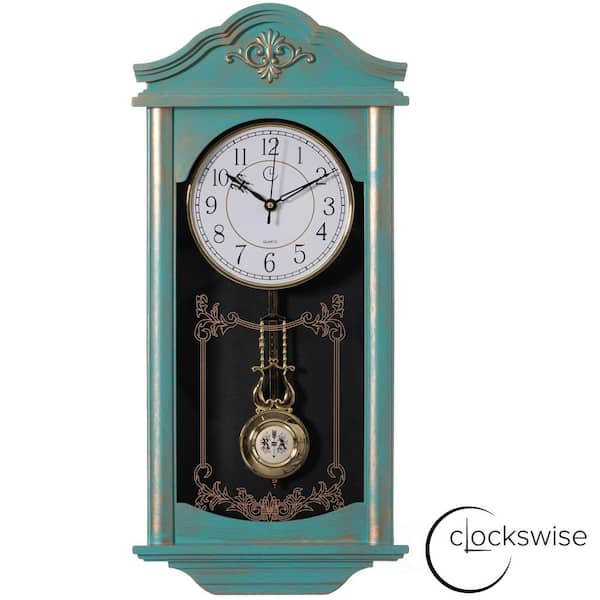This image features a vintage-style turquoise grandfather clock with parts of the color worn away, revealing underlying brass. The clock’s case is adorned with ornate, fleur-de-lis-like decoration at the top resembling a house roof, and the bottom part resembles a windowsill. The clock face is white with a brass rim, featuring black Arabic numerals and three hands, currently displaying the time as 10:10 with the second hand just past the twelve. The glass front reveals a gold pendulum below, which is embellished with letters R and A. The overall scene is set against a white background, with a black drawing of a clock in the lower right-hand corner that incorporates the word "Clockwise," where the hands of the drawn clock form the 'L' in the word. The filigree patterns and etched designs throughout add to the intricate detail of the clock.